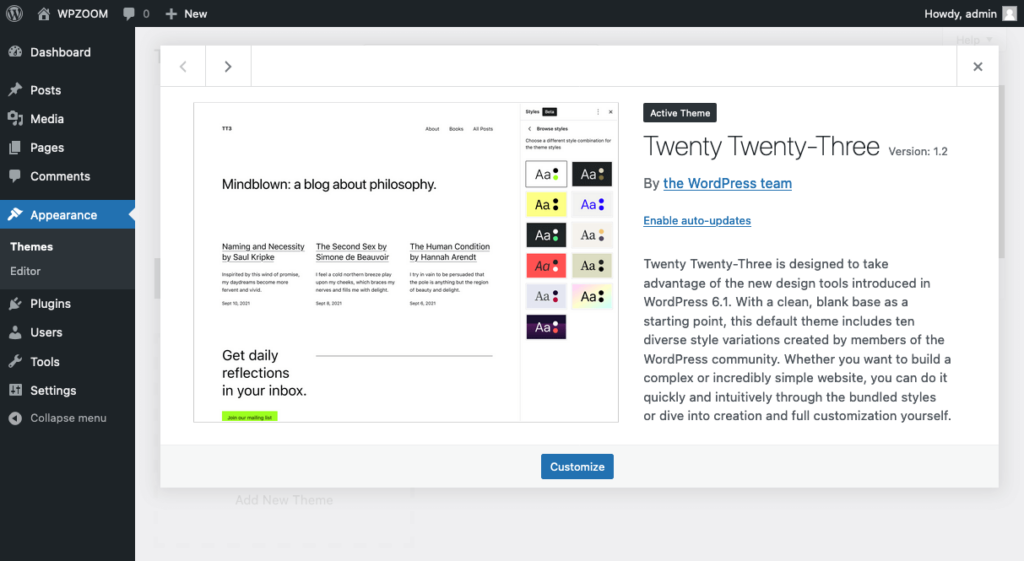A screenshot showcasing a WordPress admin dashboard with a gray background and a white content box. At the top of the box, the text "Howdy Admin" appears next to a blank profile picture outline. The sidebar menu includes: Home (with a WP Zoom icon), Posts, Media, Pages, Comments, and a highlighted Appearance section. Under Appearance, Themes and Editor are displayed with gray highlights. Additional sidebar options include Plugins, Users, Tools, Settings, and Collapse Menu.

The active theme, "2023," is detailed below, indicating version 1.2 by the WordPress team, linked in blue. An "Enable auto-updates" option is available, also in blue. The "2023" theme is described as designed to leverage new design tools introduced in WordPress 6.1, offering a clean, blank starting point. This default theme includes 10 diverse style variations contributed by the WordPress community, supporting the creation of both simple and complex websites efficiently and intuitively, whether using bundled styles or custom designs.